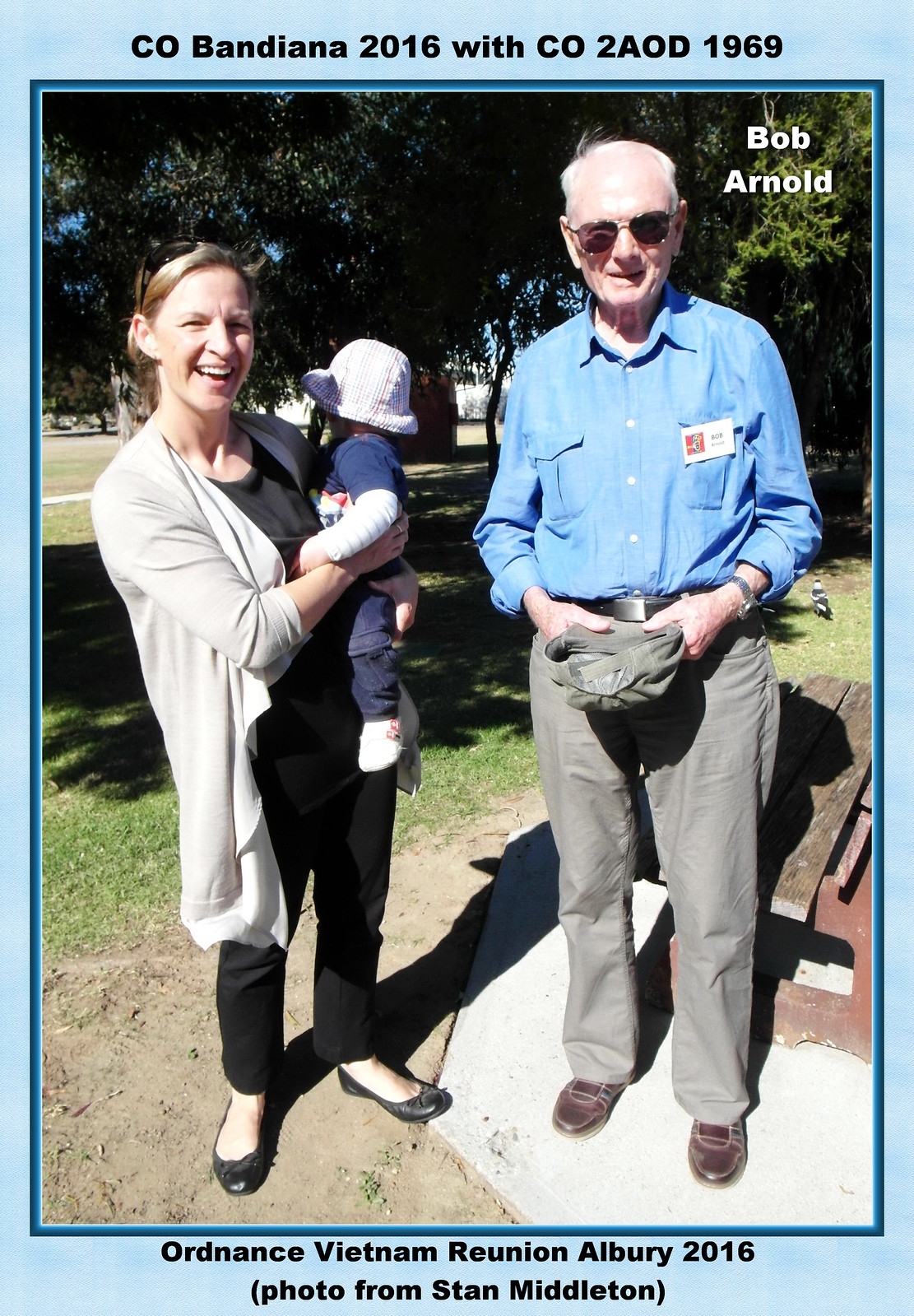This photograph captures a candid moment at the Ordinance Vietnam Reunion in Albury, 2016. On the left stands a smiling blonde woman dressed in a black t-shirt, black jeans, and black shoes, with a white long cardigan draped over her shoulders. Atop her head rests a pair of sunglasses, and she cradles a toddler who is looking away from the camera. The toddler, possibly a baby boy, wears a white hat, a blue t-shirt over a white undershirt, blue jeans, and white shoes. To the right is an older man identified as Bob Arnold, whose name appears in white letters above his head. Bob sports white hair, dark sunglasses, a blue buttoned-down collared shirt with a name tag on his left chest pocket, gray pants, and black shoes. He holds a gray hat in his hands. The setting appears to be a park with a picnic table visible in the background. The photograph is framed by a blue border with the text "CO Bandiana 2016" and "CO 2AOD 1969" at the top, and "Ordinance Vietnam Reunion Albury 2016. Photo from Stan Middleton" at the bottom.